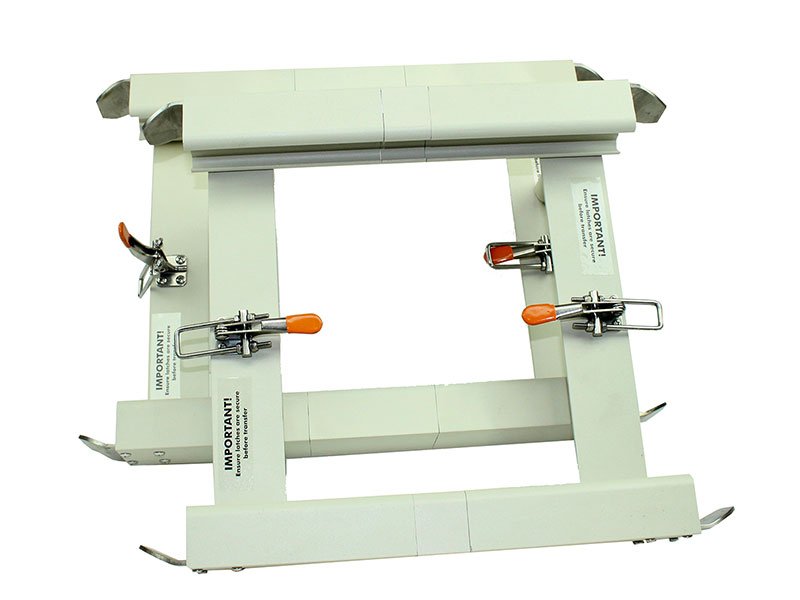The photograph captures two peculiar, square-shaped mechanical devices, each composed of a simple wooden construction painted white. Positioned with one stacked atop the other and leaning against a surface, these devices are secured with silver metal latches featuring orange handles, located on both the right and left sides. At both the top and bottom of each device, silver metal tongues protrude, while thick white metal bands run along the top. The devices also bear white stickers with black text that reads, "Important: ensure latches are secure before transfer," signifying a crucial safety instruction. The overall color scheme of the devices is predominantly white with silver metallic accents.